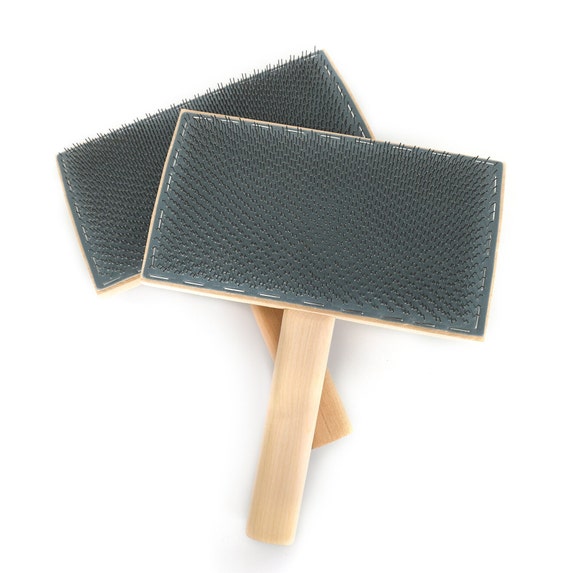The image depicts two tools with medium-length, light wooden handles, and rectangular surfaces, placed diagonally and overlapping each other on a bright white background. The surfaces of these tools are dark gray with small, needle-like protrusions and finer, hair-like fibers along the edges, giving them a spiky texture. The pad of each tool appears to be attached to the wooden block using light-colored stitching or staples around the perimeter. The tools are oriented in opposite diagonal directions, with one tool’s handle extending upward and to the right while the other’s handle extends upward and to the left. Both tools create drop shadows near their handles, indicating the bright lighting of the setting. Though their exact purpose is unclear, they resemble pet combs or hand scrubbers with a rubbery and fibrous working surface.